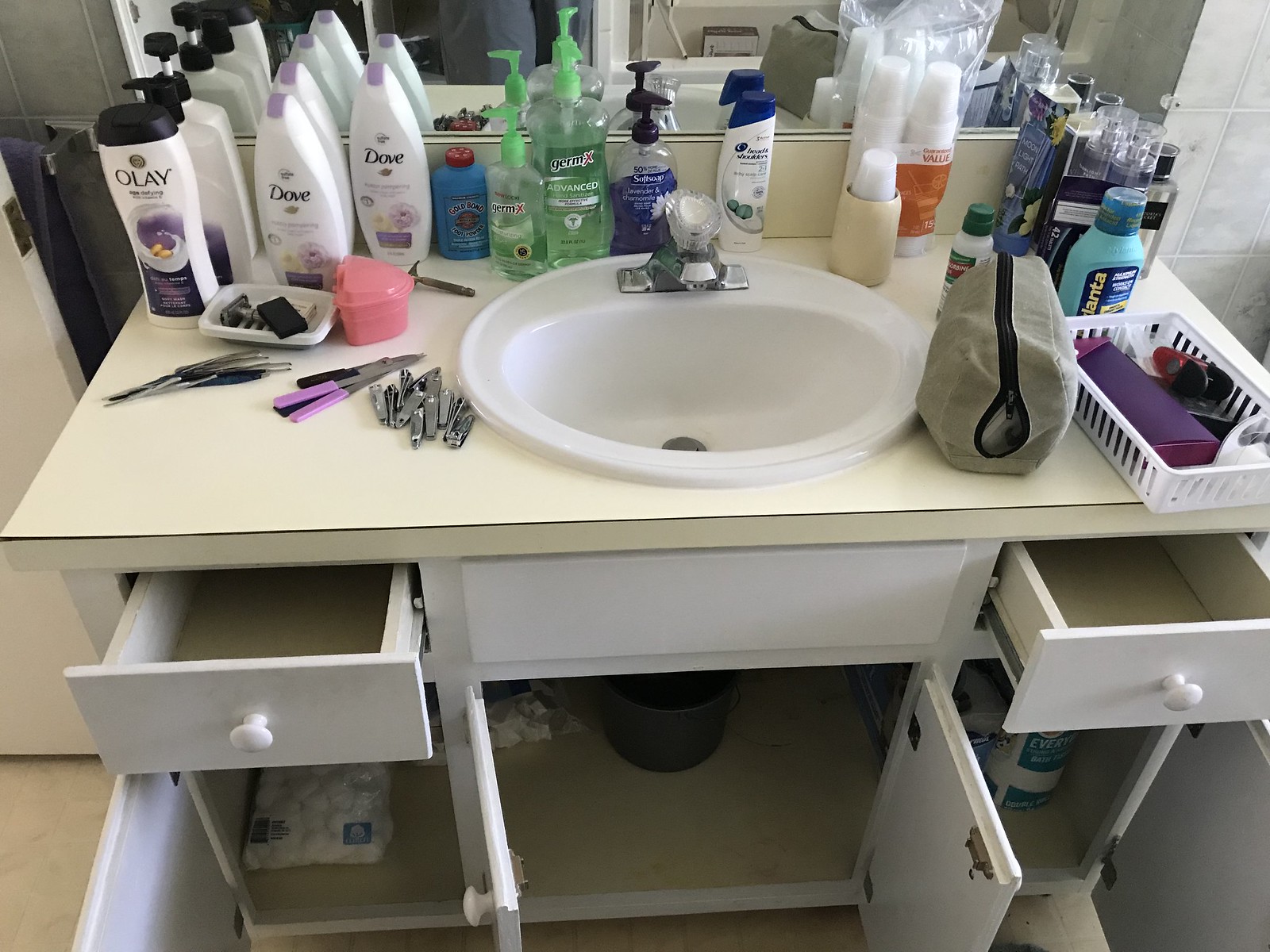This image captures a bright bathroom scene with various detailed elements. In the bottom left corner, a white towel lies on the floor. A white door is positioned on the left side of the image. Adjacent to the door, the upper left corner features a tan-grayish tiled wall with a silver towel rack holding a blue towel. 

A mirror hangs above the sink area, reflecting part of the room. In the top right corner, a light gray towel is visible. Below the counter, white cabinet doors stand open, revealing the contents within, including bags, a bucket, and various other items. The drawers are also ajar, and they have white faces with white knobs.

The countertop is a cream, off-white color, complementing the white sink and its silver faucet, which features a clear plastic handle. The sink area is bustling with personal care items, including multiple Olay body washes, nail clippers, tweezers, hand sanitizers, white plastic cups, a Mylanta bottle, and a white basket filled with additional products.